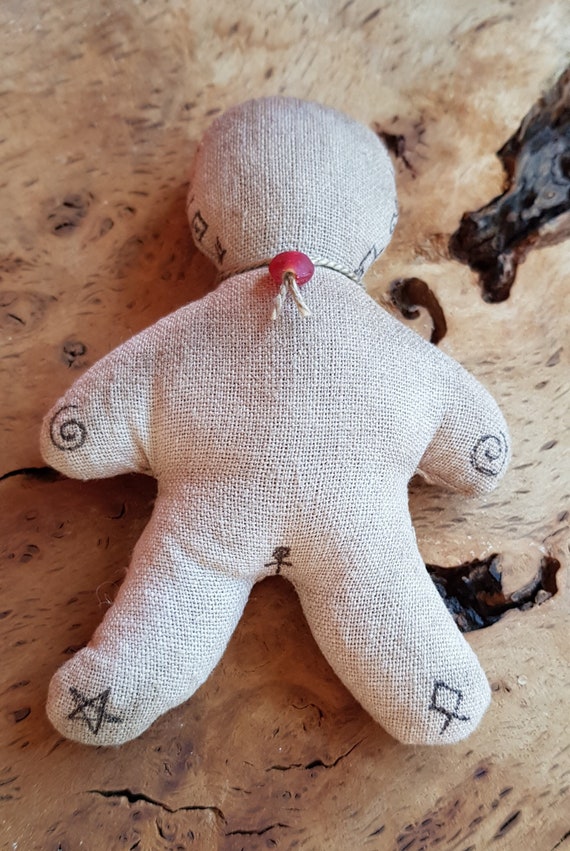The photograph showcases an intricately woven voodoo doll made of light tan burlap, sitting on a brown marble surface flecked with black. The doll, devoid of facial features, has a head, two arms, and two legs without visible fingers or toes. A black thread necklace with a red bead adorns its neck. Each hand features a swirl at the end, while unique symbols mark its legs: a star on the sole of the left foot and a diamond-like shape with two legs on the right foot. Additionally, a graphic resembling a stick figure with an outstretched arm is situated in the middle of its crotch.